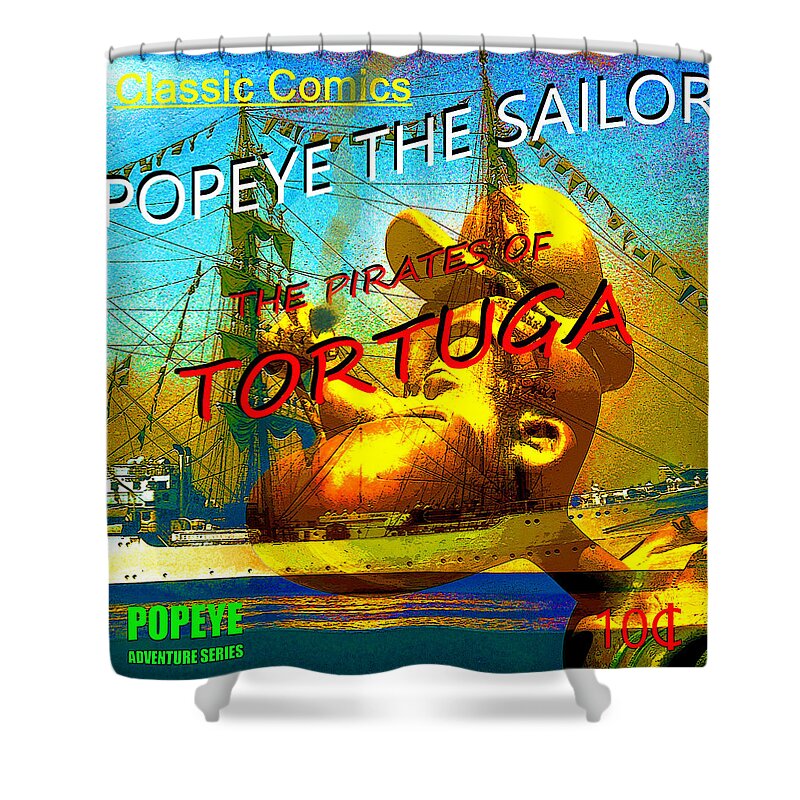This vibrant, colorful advertisement for a comic book features the iconic Popeye the Sailor Man. The top of the image boldly displays the text "Classic Comics" in a bright and eye-catching font. Below this, it prominently reads "Popeye the Sailor," and in the center, the title "The Pirates of Tortuga" suggests an adventurous storyline. On the bottom left, it mentions "Popeye Adventure Series," while the bottom right indicates the price as "Ten Cents."

The centerpiece is an image of Popeye with his eyes closed and hat tilted, against a vivid background featuring a large sailboat navigating calm blue waters under a clear blue sky. The ship, detailed with white sides, a black underside, multiple lines, and flags running through the sails, complements the superimposed image of Popeye, which predominantly features vibrant yellows. The text on the poster is in striking reds, greens, and whites, making the entire advertisement pop with vivid colors and energetic imagery. This eye-catching illustration effectively captures the adventurous spirit of Popeye in a classic comic book style.